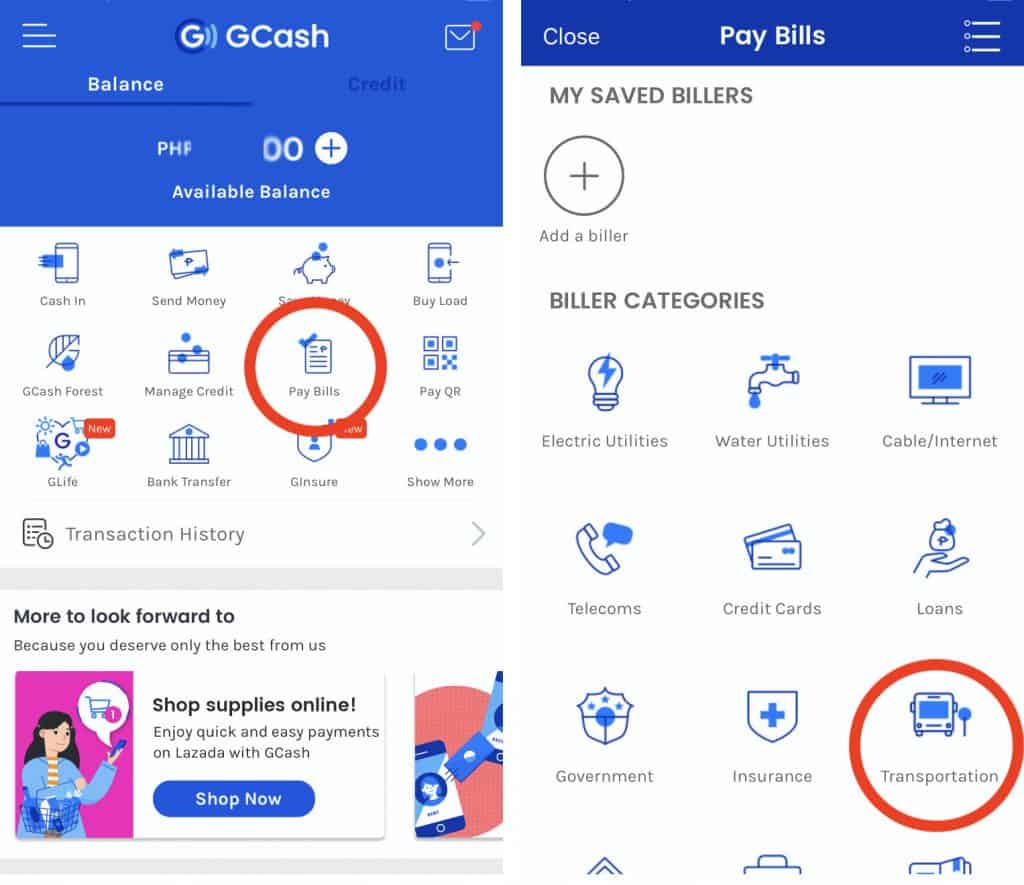Vertical split-screen image from a smart device app showcasing two distinct halves. 

**Left-Hand Side:**
- Dominated by a blue rectangular box with three lines in the upper left for more options.
- Displays the Gcash app interface featuring a small white mail icon, and various sections labeled "Balance," "Credit," and "PHF." 
- Available balance is prominently displayed, followed by various functional icons:
  - **Cash In**
  - **Send Money**
  - **A partially obscured option due to a red circle**
  - **Buy Load**
  - **Gcash for Us**
  - **Manage Credit**
  - **Pay Bills** (highlighted with a red circle)
  - **Pay QR**
  - **GLI**
  - **Bank Transfer**
  - **To Ensure**
  - **Show More**
  - **Transaction History**
- A message reads: "More to look forward to because you deserve only the best from us."
- Additional promotional content: "Shop supplies online, enjoy quick and easy payments on Lozada with Gcash. Shop now."

**Right-Hand Side:**
- Features a close button and three lines for more options at the top.
- White background titled "My Saved Bills."
- Includes an option to "Add a Biller" and categories for various services, each represented by an icon:
  - **Electric Utilities**
  - **Water Utilities**
  - **Cable Internet**
  - **Telecoms**
  - **Credit Cards**
  - **Loans**
  - **Government**
  - **Insurance**
  - **Transportation** (highlighted with a thick red circle)
- Note: The bottom three icons are partially cut off and their labels are not fully visible.